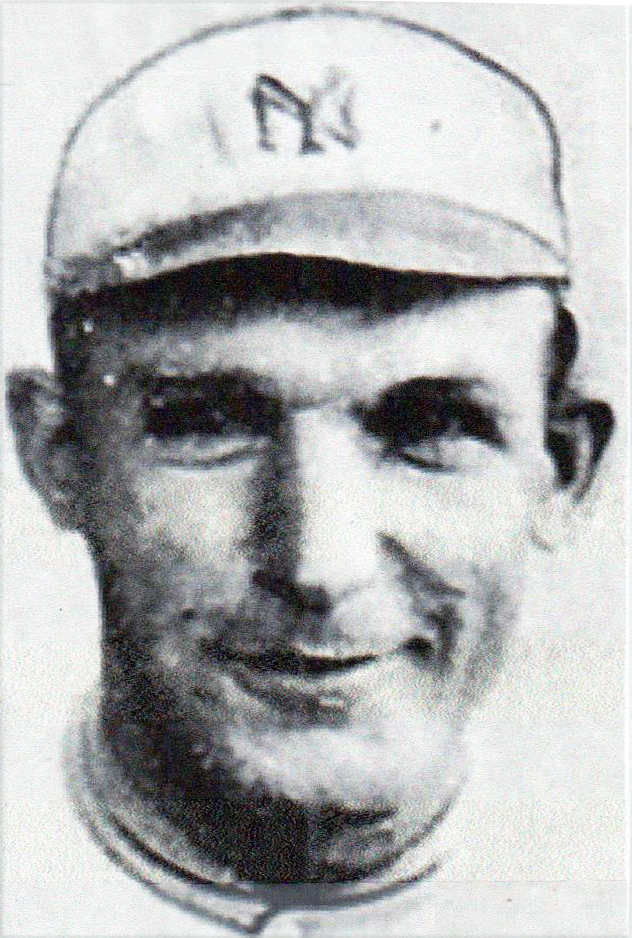This image appears to be either an old black-and-white photograph or a detailed sketch of a baseball player, likely from the early 20th century. The subject is a clean-shaven, white male in his early to mid-thirties, wearing a cap featuring the New York Yankees monogram. The cap has a notably small bill, and the player is adorned in a baseball uniform with the collar partially visible below the neck. His facial features are distinct, with notably large, pointy ears and a wide smile as he looks directly into the camera. The image is quite grainy and blurry, showing signs of either time-induced degradation or magnification. Despite the lack of identifying information about the player's name or the creator of the image, the man's joyful expression and the historic styling hint at his prominence in New York Yankees history.